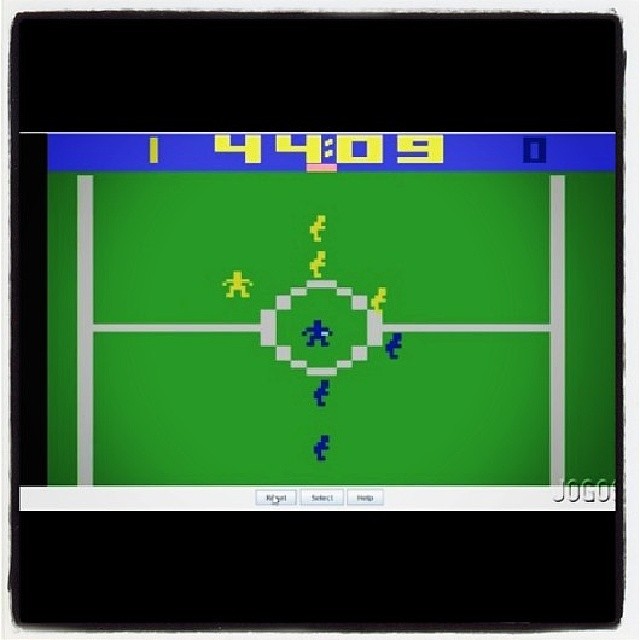A nostalgic screen capture depicting a rudimentary soccer video game. The image is framed by plain black bands at the top and bottom, while the game itself occupies a wide horizontal strip in the center. The game's graphics are minimalist, showcasing a green field with simplistic gray lines marking the scoring zones. On the field, there are eight highly pixelated and basic figures — four in yellow uniforms and four in blue. The player in the center, dressed in blue, is characterized by a white dot indicating possession of the ball. Above the gameplay area, an unobtrusive scoreboard displays the current status: Yellow team leading with a score of 1, blue team trailing with 0, and the game clock at 44:09.